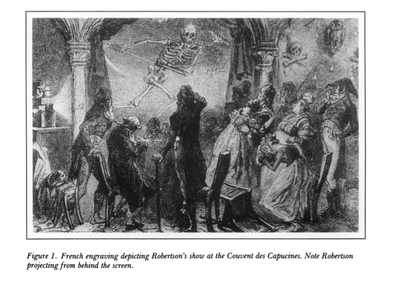This is a detailed black and white French engraving titled "Figure One," depicting Robertson's show at the Covenant de Capucino. The scene captures a Revolutionary-era audience dressed in Napoleonic attire, some in shock and consternation as they witness a skeleton dancing, projected from behind a screen. The faces of the audience are obscure, with some people seemingly flying backward in fear, and overturned chairs adding to the chaotic atmosphere. Details in the foreground include a stick-like dog and a skull and crossbones hanging from a tree, while on the left side, a man with a light projector is shown creating the eerie spectacle.